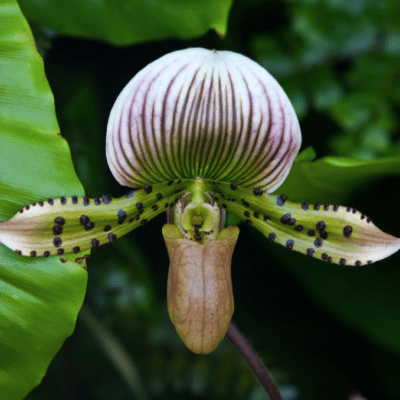This square photograph captures an exotic and peculiar flower set against a backdrop of dark, blurred foliage. Dominating the background towards the left is a single protruding leaf of lighter green color, providing contrast to the overall scene. At the center, the flower features an intriguing arrangement: above, a large, curved petal with a white base, highlighted by striking off-purple or magenta vertical stripes extending outward. This petal appears voluminous and cotton-like. Below, two greenish petals stretch horizontally, extending to the left and right, both adorned with distinct black or dark brown spots. Completing the composition is a downward-facing, tube-like structure with a peach-brown, veiny texture, resembling a pitcher or small glass. Overall, this detailed image portrays the flower in a lush, forest-like setting, emphasizing its unusual beauty.